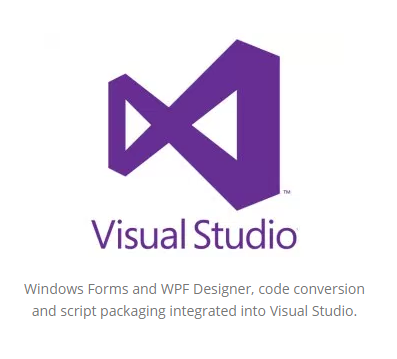In the image, the design is clean and minimalistic with a white background. Dominating the center is a logo resembling a stylized bowtie, tilted slightly to the left; the bowtie shape is purple with white interiors. Directly beneath the logo, "Visual Studio" is written in bold purple text. Following this, in smaller gray text, the description reads: "Windows Forms and WPF Designer, code conversion, and script packaging integrated into Visual Studio." This succinctly conveys the advanced features integrated into Visual Studio.